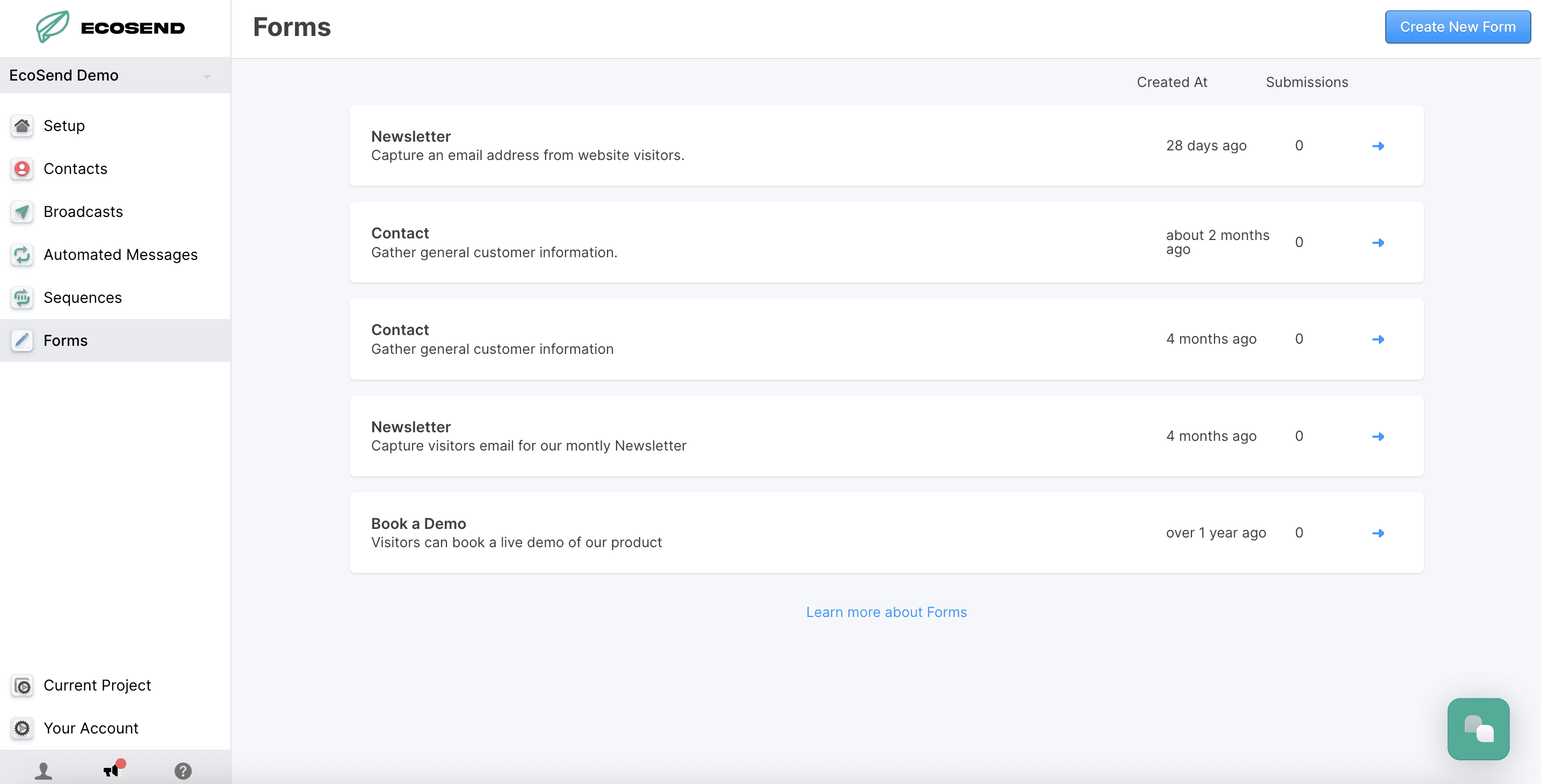The image is a screenshot of the Ecosend desktop application/website, showcasing its user interface. It features a clean, white background dominated by text elements. The layout includes a navigation column on the left-hand side, where the "Ecosend" name appears prominently in bold black text at the top. Adjacent to the name is a small logo, which resembles a green line drawing that could be interpreted as either a paper airplane or a leaf.

Within the navigation column, several categories are listed in sequence: Ecosend Demo, Setup, Contacts, Broadcast, Automated Messages, Sequences, and Forms. The Forms category is currently selected. The right-hand section of the interface presents a detailed list of different forms available in the application. These forms include Newsletter, Contact (appearing twice), another Newsletter, and Book a Demo. Each form entry displays additional information, such as the date of creation and the number of submissions received.